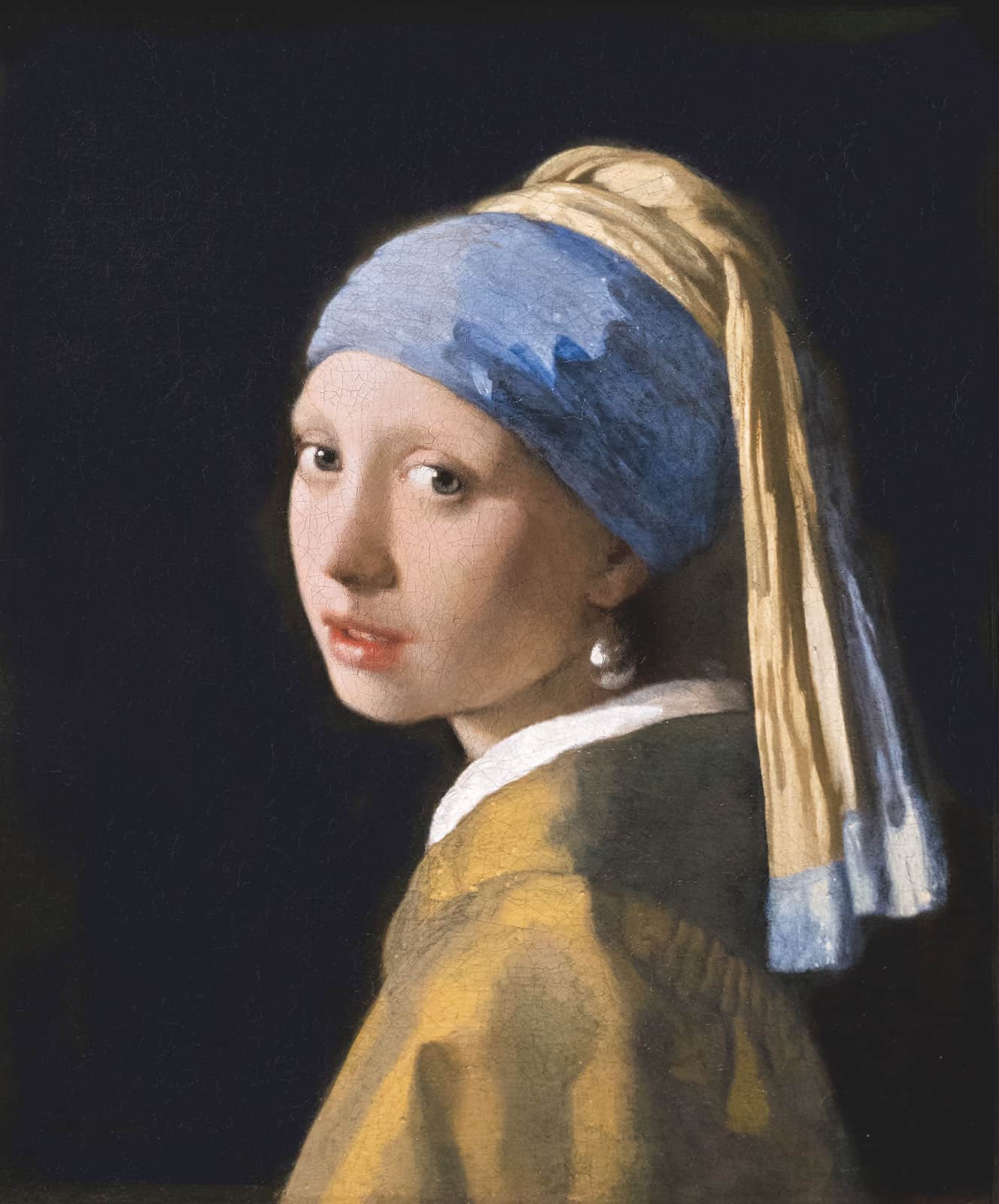This striking painting depicts a young woman with a serious yet curious expression. She is adorned with a distinctive blue headscarf that wraps around her head, with a gold section that drapes down to her shoulders, creating a contrasting and eye-catching element. Her thick headband, or turban, adds a sense of elegance to her appearance. The young lady features red lipstick and wears large silver earrings, emphasizing her delicate and fair skin. Her eyes, which are either green or brown, contribute to her inquisitive and direct gaze. Her attire consists of a white shirt beneath a beige and brown garment, which some describe as a coat or jacket with burnished tones. Set against a pitch-black background, the figure stands out vividly, particularly highlighted by the light blue and gold of her headscarf. While the painting lacks any text or signature, its composition and detail make it reminiscent of the famous "Girl with a Pearl Earring," showcasing a beautiful and captivating portrait.